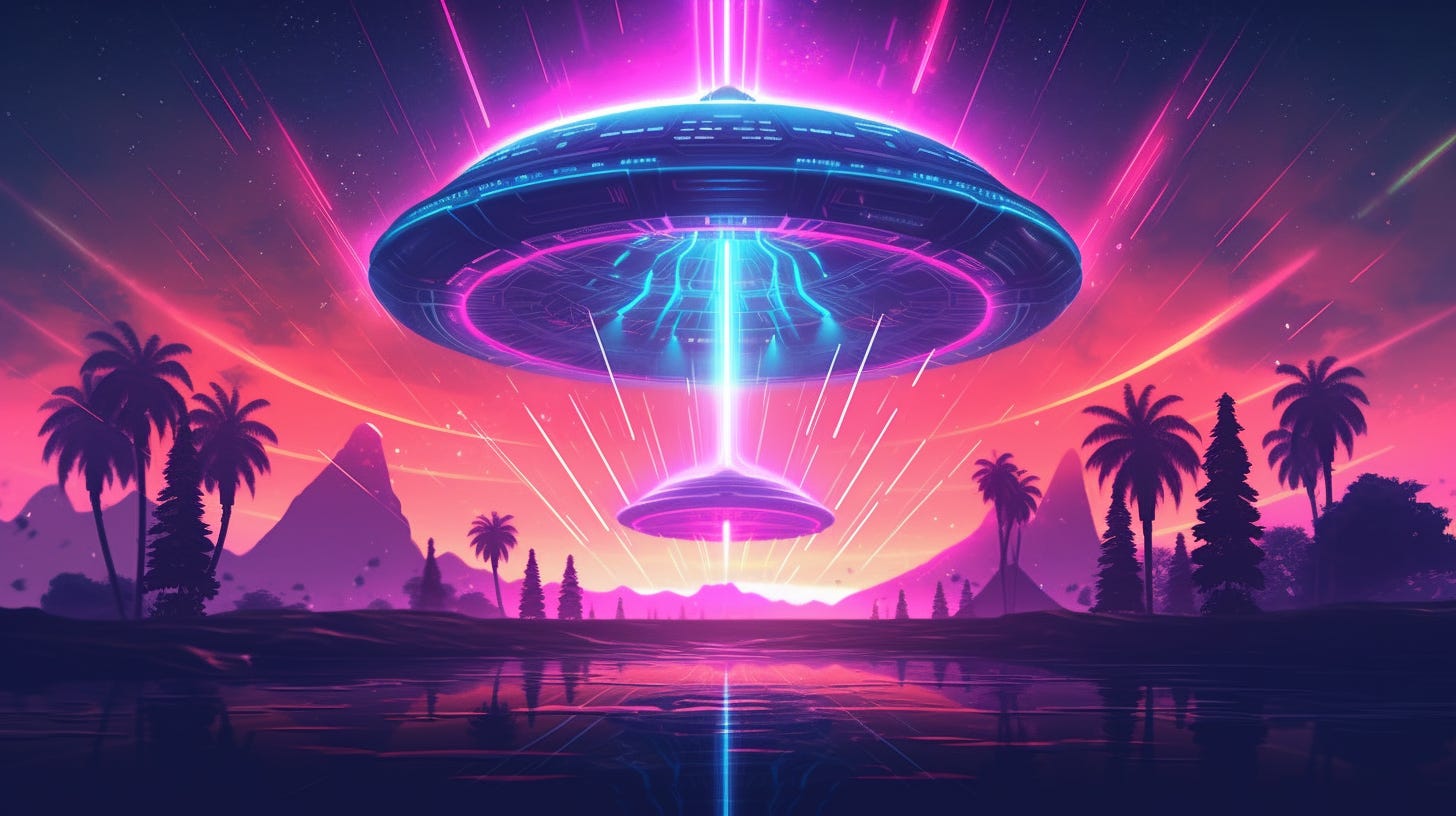The computer graphic artwork depicts a vivid, surreal desert scene, likely set in a location reminiscent of Egypt, with a dramatic sky illuminating the landscape in purples, pinks, and blues. Dominating the scene is a large, traditional UFO-shaped mothership with a glowing, red-purplish halo, emitting bolts of electric currents down to a smaller, circular UFO directly below it. The smaller craft is bathed in shades of pink and mirrors the mothership's shape and luminosity. This dynamic interplay of light and electricity between the crafts lights up the shiny ground, creating vivid reflections that contrast against the dark, wet surface. Surrounding the UFOs are tall, jagged mountaintops, some with peaks and others resembling Christmas trees, interspersed with iconic palm trees, all contributing to the artwork’s otherworldly atmosphere. The overall scene evokes the aesthetic of a science fiction movie, blending imaginative elements with a colorful, neon-like palette.